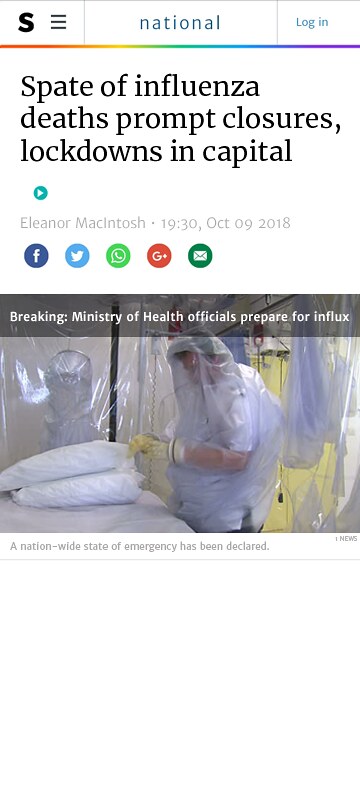This image is a detailed screenshot of a webpage from a news website, presumably Salon, recognizable by the capital letter "S" in the top left corner. The "S" is followed by three horizontal lines indicating a clickable drop-down menu. At the top center, the word "National" is prominently displayed, while the top right features a blue "Log In" button with a rainbow-colored horizontal line underneath.

The article's headline reads, "Spate of Influenza Deaths Prompt Closures, Lockdowns in Capital." Below the headline, it lists the author as Eleanor McIntosh with the date October 9, 2018. There are circular social media icons for Facebook, Twitter, email, Google, and a phone logo, facilitating easy sharing of the article.

An image at the bottom features a person in full protective gear, including plastic gloves, standing in a sterile, transparent-curtained area near a bed with two pillows. A caption below the image states, "Breaking: Ministry of Health Officials Prepare for Influx," and notes that a nationwide state of emergency has been declared.